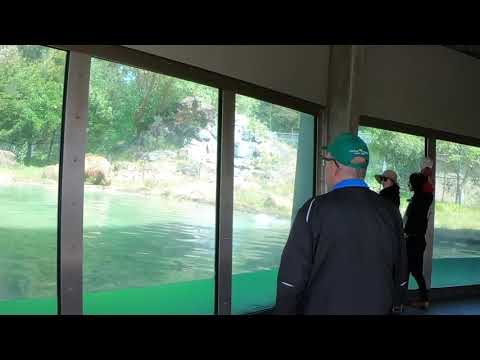The image is set within a room bordered by long, black horizontal bars at the top and bottom, giving a framed effect. Inside the room, there are three people standing in front of a wall dominated by tall windows with steel brackets. Through these windows, there is a view of knee-high water, vibrant in shades of green and blue-green, and a rocky hill with trees in the background. The man front and center is wearing a green ball cap, glasses, a blue collared shirt, and a black jacket. Behind him stand two women: one in a sun hat, sunglasses, and a black coat, and the other in dark clothing. All three individuals are looking out at the serene aquatic scene, reminiscent of an aquarium exhibit, although no animals are visible in the water.